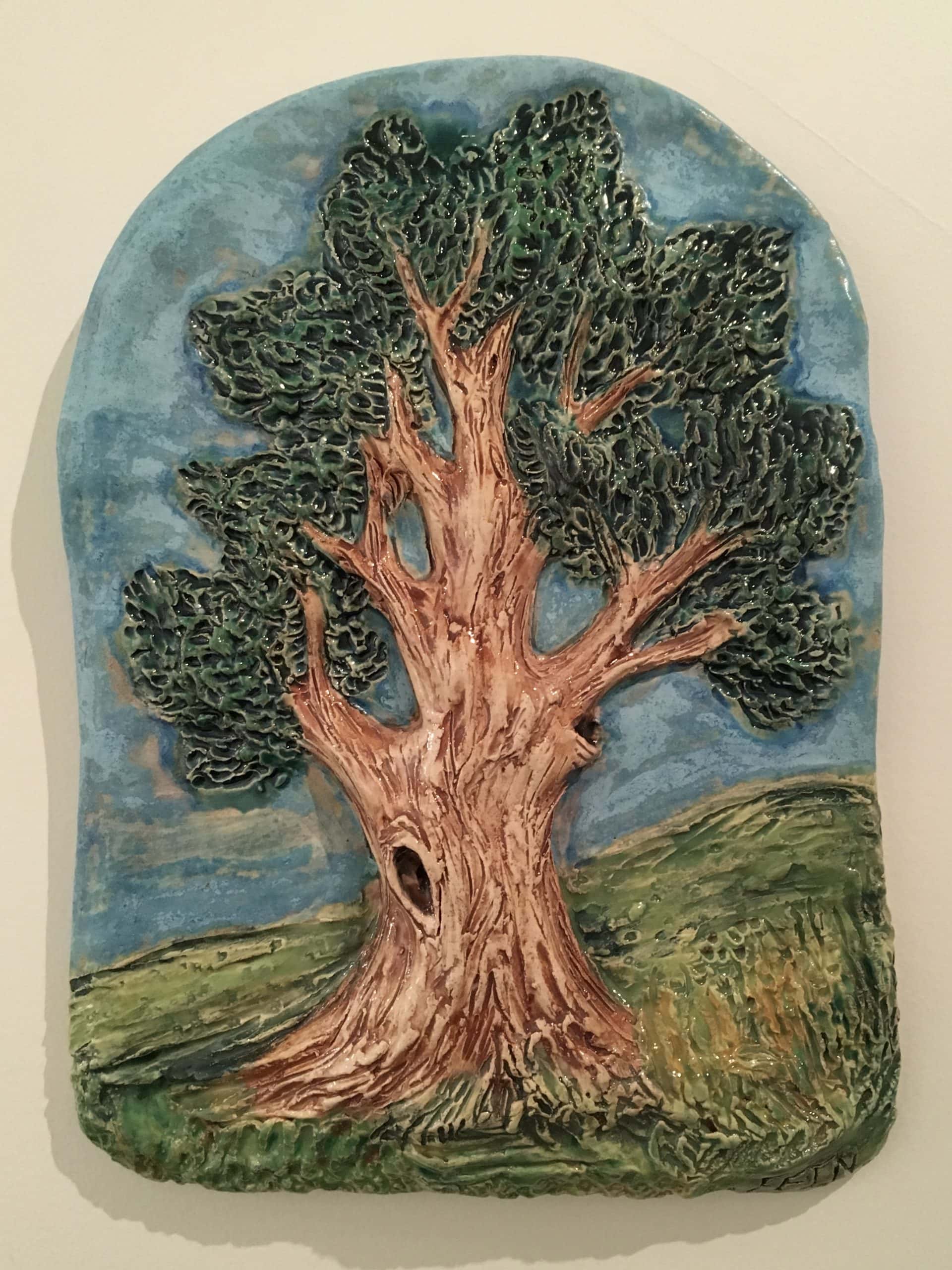The artwork is a porcelain or ceramic piece that hangs on a wall, depicted in a shape reminiscent of a stone tablet or a tombstone. It features a highly detailed, three-dimensional embossed scene of an old knotted tree with a wide base and thick branches, indicating its age. The tree trunk is light brown and includes a large hole, adding to its character. The foliage is dark green with a sponge-like texture and extends across the entire width of the piece. This tree is situated in a grassy field with a green hill behind it, under a blue sky. Muted colors and shadows suggest it's displayed indoors, with no text present on the piece. To the right, there are pussy willows and what appears to be yellow flowers, adding more depth and color to the artwork.